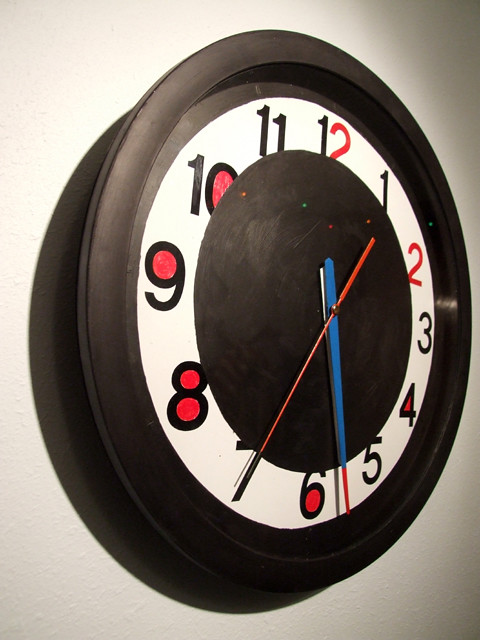This photograph features a wall-mounted clock at a slight angle on a white wall. The clock itself is notably tilted to the right within the frame. It has a thick, black plastic border, which contrasts sharply with its white face. The clock's numbers are an alternating mix of black and red, with the 12 displayed in black, while the 2, 4, 6, 8, 9, and 10 are in red. The clock hands are colored red and blue, adding a splash of additional color. The central hub of the clock is a black section, seemingly covered, potentially also made of plastic. A noticeable shadow of the clock falls to the left, adding depth to the image.